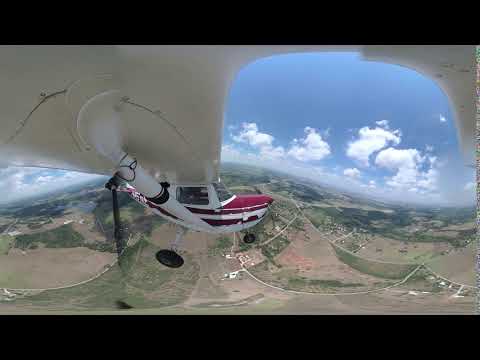The image showcases a panoramic view captured from a camera attached to the underside of the right wing tip of a small, red-and-white propeller airplane in flight. The aircraft, which has its wings positioned above the cabin, is prominently situated on the middle left side of the image. The propeller is visible at the front, along with wheels that are extended rather than retracted—the larger black wheel at the back and a smaller one beneath the front engine. The sky, visible on the right and partially on the left, is a clear blue adorned with puffy white clouds. Below, there's a rural landscape featuring a patchwork of dry, light brown fields and areas highlighted with green representing forests or trees. The photograph is bordered by thick black strips at the top and bottom, framing this detailed scene.